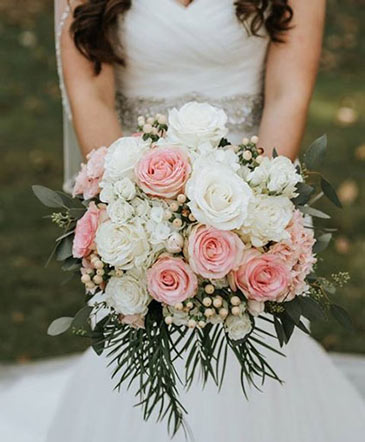Gazing down from above, the bride cradles an exquisite bouquet, her elegant crisscross wrap style dress subtly embracing her form. Her long, wavy brown hair cascades just past her shoulders, complementing her bare arms that extend gracefully, revealing tender elbow creases and part of her upper arms. The dress, adorned with intricate silvery floral beadwork around her waist, cascades into a flowing skirt which transcends into a delicate train. She's positioned on a verdant lawn, enhancing the natural charm of the setting, though the emphasis remains intimately on her bouquet. 

The bouquet, a harmonious blend of pale pink and white roses, evokes a sense of timeless romance. Each bloom, full and peony-like, is meticulously arranged among smaller rose buds and delicate baby's breath. The bouquet’s lush composition is framed by graceful, slender leaves and bluish ovate foliage, resembling eucalyptus, adding depth and texture to the arrangement. This rounded, voluminously designed bouquet, with at least a half dozen of both pink and white roses, exudes a meticulous beauty, symbolic of the love and care inherent in this moment.